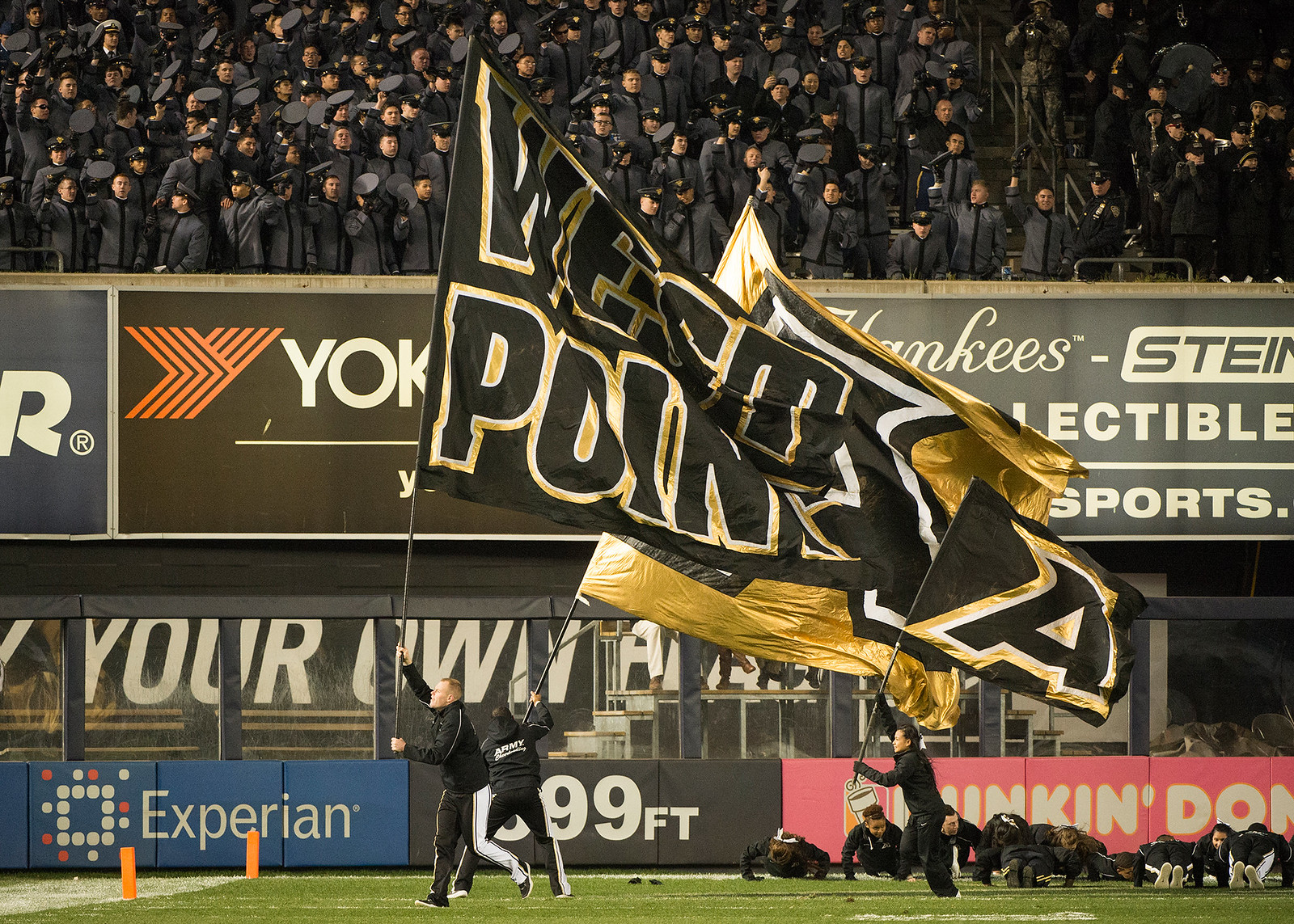In this color photograph taken at the West Point Military Academy sports field, we see a vibrant display of military precision and pride. The green turf of the football field is the stage for the central action—a young man dressed in a black sweatsuit running across the field, prominently carrying a large black-and-gold flag that boldly reads "West Point." Accompanying him are two other men, also in black sweatsuits, holding smaller and medium-sized flags. 

To the right, a row of men in athletic gear are performing push-ups, demonstrating physical discipline. The stands in the background are filled with hundreds of West Point cadets, all dressed in gray uniforms and some wearing caps. These cadets stand in formation, creating a sea of military uniformity, as they watch their flag being paraded across the field. Banners and advertisements adorn the barrier wall around the field, with visible names like Dunkin, Experian, and various collectibles and sports-related companies.

The overall atmosphere suggests a ceremonial or celebratory event, showcasing both the physical prowess and the collective spirit of the West Point cadet corps.